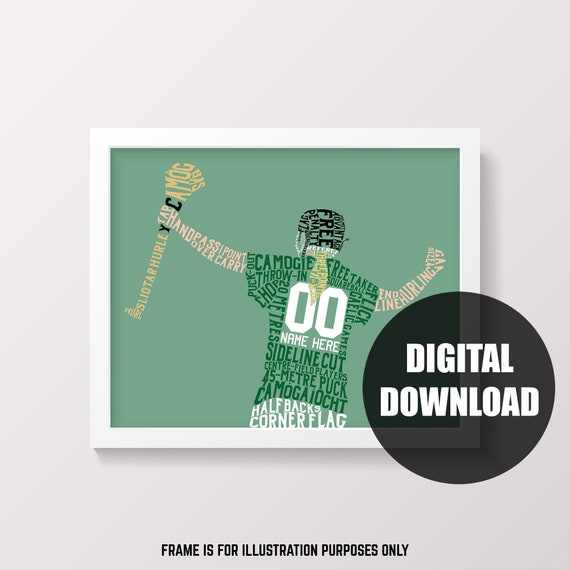The image is a detailed graphic piece displayed on an off-white, wall-like background. It features a central, rectangular artwork with a white frame, set against a light pastel green backdrop. Dominating the center is the back view of a lacrosse player – depicted as a woman with a ponytail – holding a sports instrument in the left hand and raising the right hand in a fist. This figure is uniquely illustrated with words in various colors representing different body parts: a peach-colored font for the arms, dark green for the jersey, and white for the shorts. The jersey features the number "00" in white with the text "Name Here" below it. The helmet on the player's head bears the word "free."

At the bottom of the framed artwork, in small black font, is the disclaimer "FRAME IS FOR ILLUSTRATION PURPOSES ONLY." Additionally, in the bottom right quadrant, there is a large black circle with white text reading "Digital Download," partially enveloped by a semi-transparent dark gray or black watermark. Throughout the image, words like "sideline" and "out" are meticulously incorporated into the design, adding to the intricate detailing of the artwork.